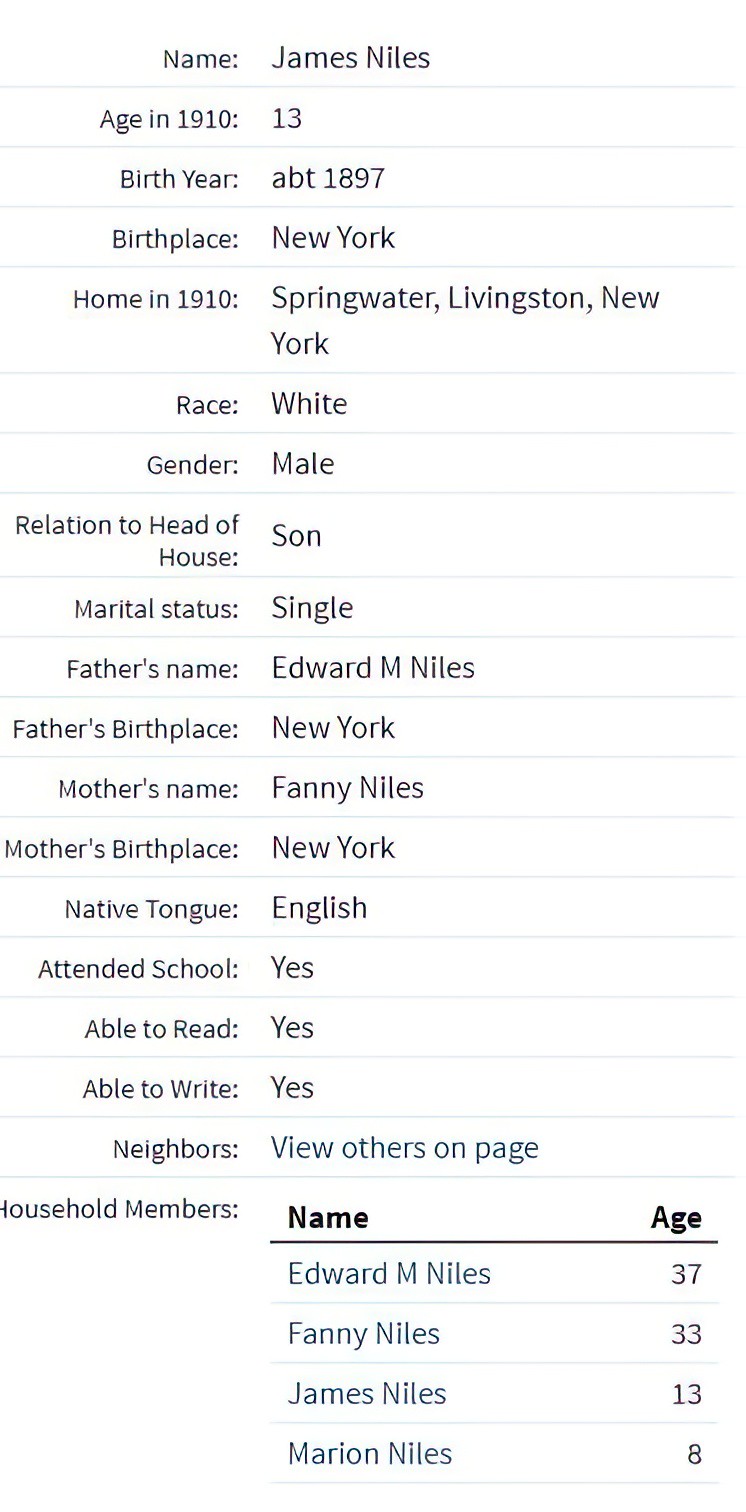This image is a rectangular, informational form with a white background and black text, separated by thin gray horizontal lines. It details the personal information of an individual named James Niles. The text reads as follows: 

- **Name:** James Niles
- **Age in 1910:** 13
- **Birth Year:** About 1897
- **Birthplace:** New York
- **Home in 1910:** Springwater, Livingston, New York
- **Race:** White
- **Gender:** Male
- **Relation to Head of House:** Son
- **Marital Status:** Single
- **Father's Name:** Edward M. Niles
- **Father's Birthplace:** New York
- **Mother's Name:** Fanny (or Fannie) Niles
- **Mother's Birthplace:** New York
- **Native Tongue:** English
- **Attended School:** Yes
- **Able to Read:** Yes
- **Able to Write:** Yes
- **Neighbors:** View others on page
- **Household Members:**
  - Edward M. Niles, age 37
  - Fanny Niles, age 33
  - James Niles, age 13
  - Marion Niles, age 8